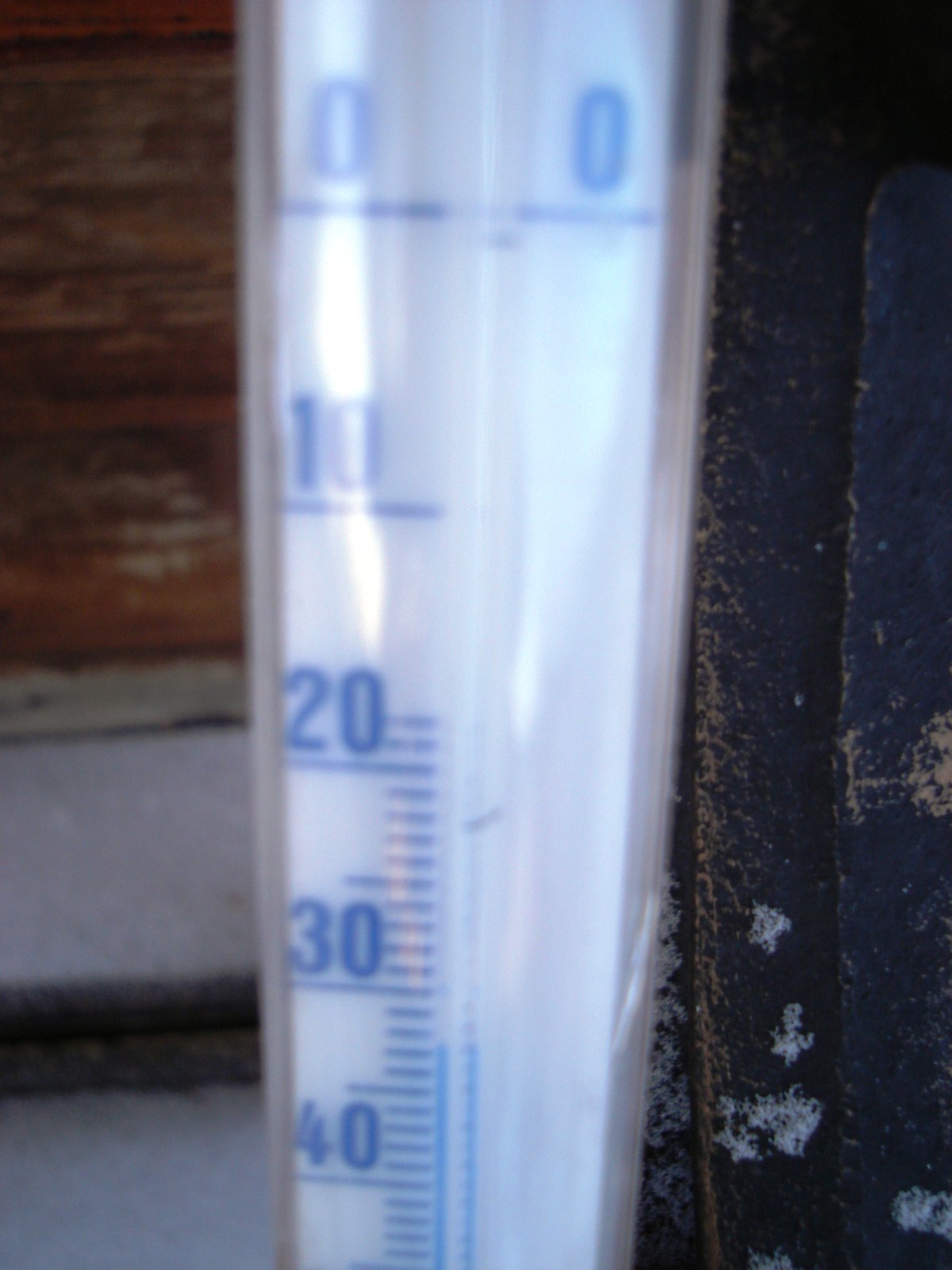The image is a very close-up and somewhat blurry photo of a clear plastic thermometer with blue numbering and markings in increments from 0 to 40 degrees. A partial segment of the thermometer is in focus, with a hint of blue liquid visible. There is a noticeable glare from light reflecting off the thermometer's surface. The blurred focal point of the image includes a black metallic frame situated to the right. Behind the thermometer, there is horizontally aligned wood paneling and a wide, white baseboard at the bottom, possibly part of a house or similar structure. The setting appears to have a gray floor and may also include some steps in the background. The thermometer is likely used to check ambient temperature, though the exact reading is indiscernible from the image.